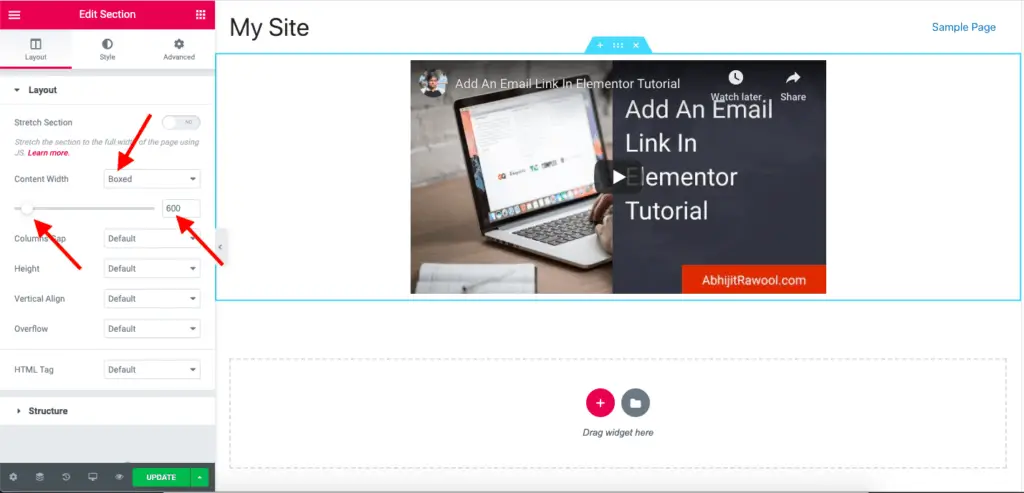Image Description: The image showcases a website management control page with various application and resource settings. At the top left, there is a red button with white text that reads "Edit Selection." To its left, there is a three-bar menu icon. Below this section, the page background transitions from white to gray.

Within this section, there are layout options labeled as "Style" and "Advanced." The layout text is grayed out, indicating it is inactive. A prominent red arrow is superimposed on the image, pointing towards a widget box located on the right side of the content width, which is set to "Based."

Further down the page, another superimposed red arrow points to a slider bar, highlighting adjustments near the bottom left. The slider's value is set to 600. Below the slider, several layout settings are listed, including "Columns: Default," "Height: Default," "Vertical Align: Default," "Overflow: Default," and "HTML Tag: Default." These settings are also in gray text, implying default or inactive status.

At the bottom of the image, there is a video link titled "Elementor Tutorial"—the video appears to be hosted on YouTube, indicated by the familiar play button icon and a gray, unplayed progress bar.